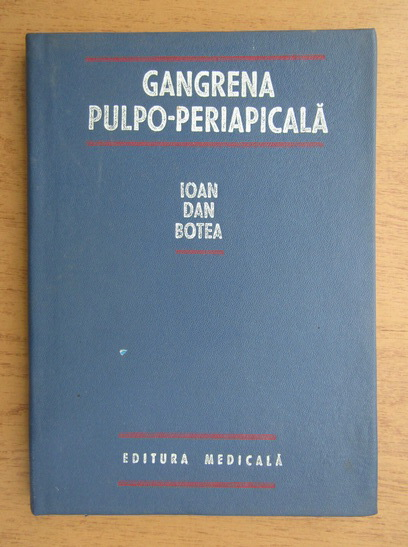The image depicts a navy blue paperback book with white text and red demarcating lines. At the top center of the cover is the word "Gangrena," followed by "Pulpo Puripasa Pakala." Below that, centrally positioned, are the names "Ayoan Dan Botea," and at the bottom center, "Editura Medicala" is inscribed. Each of these text sections is separated by horizontal red lines. The book is resting vertically on a brown wooden desk, suggesting a simple, possibly academic setting. The overall foreign text and medical terminology allude to the book being some form of medical literature.